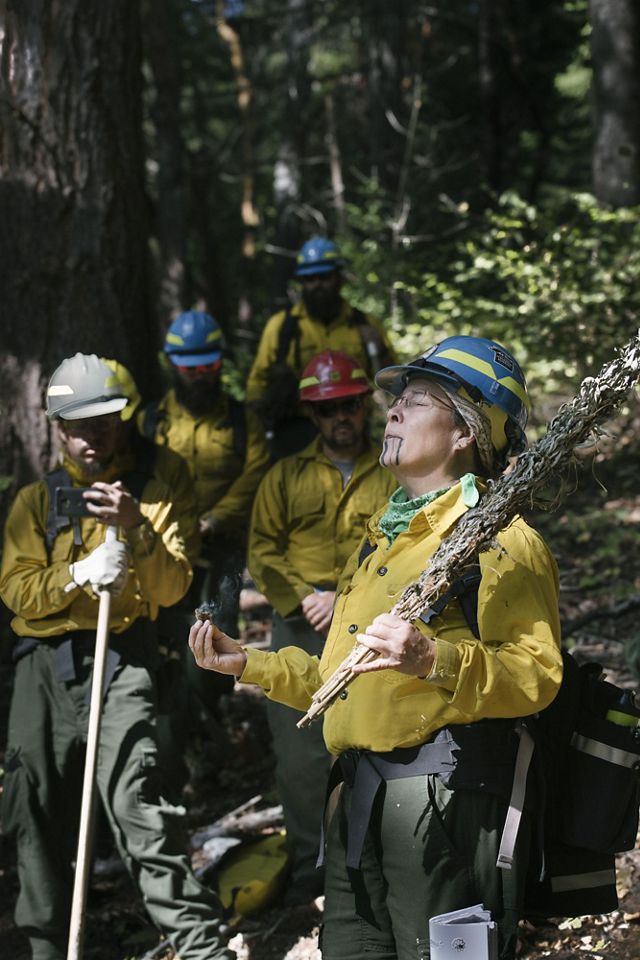In the midst of a dense, dimly lit forest, a work crew of five individuals stands out against a backdrop of towering tree trunks and lush green leaves. Each person is outfitted in long-sleeved yellow shirts and dark pants, and they're all donning hard hats: three in blue with a yellow stripe, one in red, and another in white. Two men sporting beards and sunglasses are among them, alongside another man equipped with a harness that suggests gear for forest navigation or heavy lifting. 

But the focal point of the image is an older woman in the foreground, brightly illuminated and facing the sunlight. Her blue-and-yellow striped hard hat adds to her authoritative presence, complemented by her firm grip on a large, rough-textured wooden stick that converges into a sharp point. Her eyes are closed, and peculiar black marks reminiscent of ink or face paint are spilling from her mouth down her chin, as if she had consumed something causing this odd effect. In her left hand, she holds a small, indistinct object, possibly a plant. The remaining workers, slightly blurred in the background, observe her with a mix of curiosity and attention, highlighting her as a central figure in this enigmatic woodland scene.